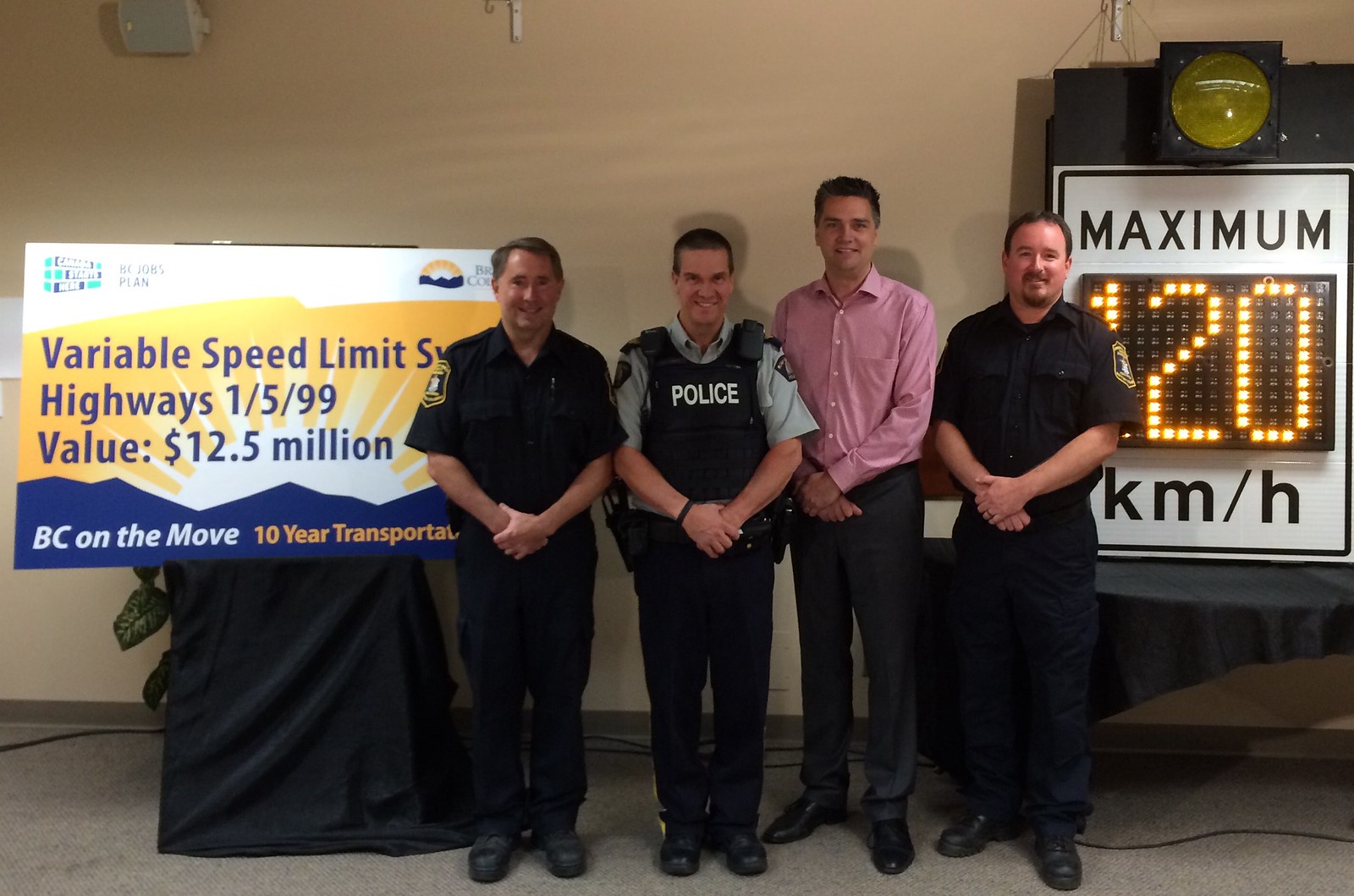In the center of this color photograph are four adult men, arranged side by side and facing directly at the camera. Three of them are in various police uniforms, while the fourth is dressed in civilian attire. The man on the far left is a Caucasian male with short brown hair parted neatly from left to right. He wears a black uniform adorned with a badge on his left arm and stands with his hands folded over his stomach. 

Next to him, also dressed in police attire, is a man with a black vest labeled "police" over a gray shirt. He has short black hair and looks directly into the camera. The third man is the tallest of the group, sporting wavy black hair. He is dressed in formal business attire, featuring a pink button-down Oxford shirt and dark pants. 

The final man on the far right is clad in a black uniform similar to the first man’s, with a badge on his right arm. He has a mustache and goatee, and he too has his hands resting in front of him.

To the right of this group stands a large digital speed limit sign that reads "MAXIMUM 120 kilometers per hour" in illuminated text. On the left side of the frame is a banner that details a transportation initiative. The banner reads "Variable Speed Limit System Highways, 1/5/99, Value: 12.5 million, BC on the Move, 10-year Transportation." The backdrop and positioning of these elements suggest a professional or official setting, possibly a press event or a formal announcement related to traffic or transportation.